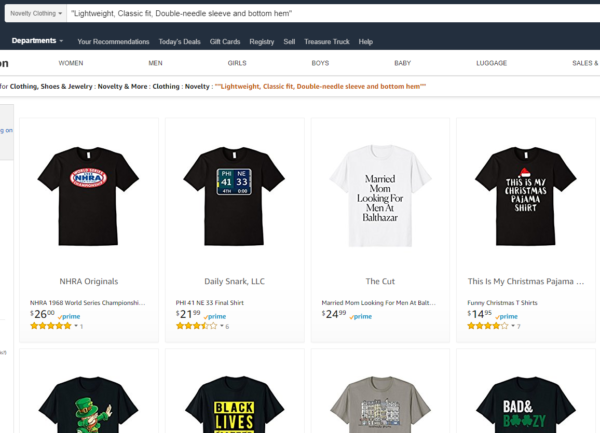This is a screenshot of an Amazon storefront, specifically for a novelty clothing store. The top of the page features a header that reads "Novelty Clothing" and includes a search box with preset filters: "lightweight," "classic fit," "double-needle sleeve," and "bottom hem." Just below, navigation categories are neatly displayed for easy browsing, including options like Women, Men, Girls, Boys, Baby, Luggage, and Sales.

Eight t-shirts with different graphic designs are displayed in a grid format. The top row comprises four short-sleeve black t-shirts, each with distinct pricing and reviews. The t-shirt on the upper left features an "NHRA 1968 World Series Championship" design, boasts a 5-star rating based on one review, and is priced at $26. The next three black t-shirts in the top row are priced at $21.99, $24.99, and $14.95, respectively. All t-shirts display the Amazon Prime logo, indicating fast shipping options.

The bottom row showcases another set of t-shirts: two black, one white, and one medium-light gray. Due to the cropped nature of the screenshot, the prices for these t-shirts are not visible, nor are any additional details beyond the upper portion of the products. The overall design and layout are user-friendly, capturing the essence of Amazon's recognizable interface.